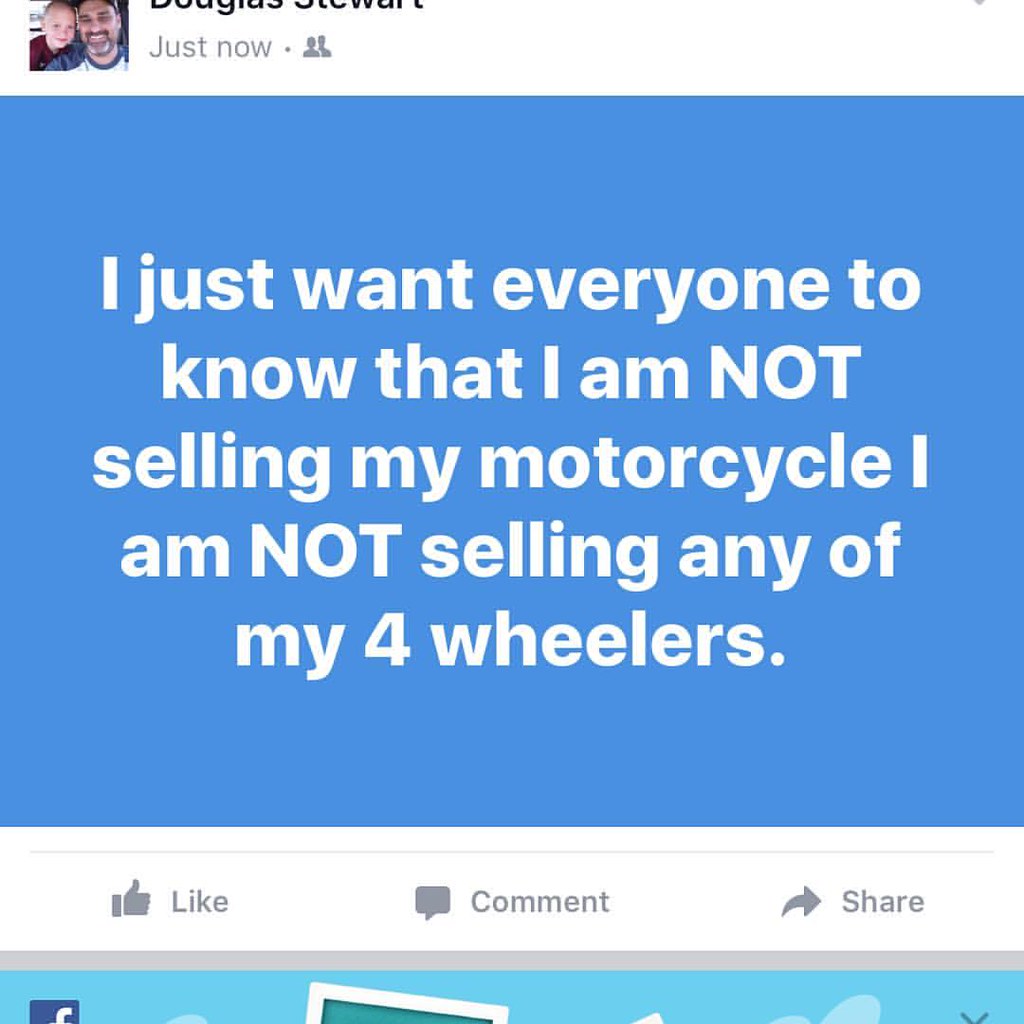The image is a screenshot of a social media post, likely from Facebook, made by a man whose partially visible name might be Douglas Stewart. His profile picture features himself with a child. The post, set against a blue background with white text, states emphatically: "I just want everyone to know that I am NOT selling my motorcycle. I am NOT selling any of my four-wheelers," with "NOT" being capitalized for emphasis. Below the post, the usual Facebook options for Like, Comment, and Share are visible, though no interactions have been made yet as it appears to have been posted recently.